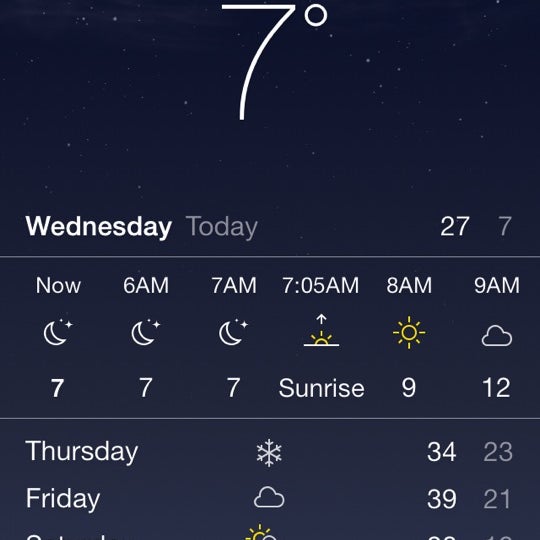The image depicts a weather app interface set against a backdrop of a starry night sky. The app displays the current temperature of 7 degrees as well as today's date, indicating it is a Wednesday. The forecast for the day includes a high of 27 degrees and a low of 7 degrees. 

Detailed hourly temperature information shows:
- 6:00 AM: 5 degrees
- 7:00 AM: 7 degrees
- 8:00 AM: 7 degrees
- 9:00 AM: 9 degrees

Additionally, upcoming weather conditions for Thursday and Friday are provided:
- Thursday: A mix of snow and rain is expected, with a high of 34 degrees and a low of 23 degrees.
- Friday: The forecast includes a high of 39 degrees and a low of 21 degrees.

All text is rendered in white, contrasting effectively with the black or starry sky-colored background, ensuring readability.